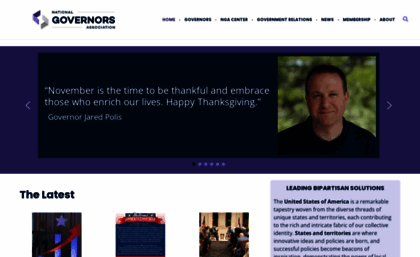The image depicts a national governor's website interface. Positioned across the top, from the middle to the right-hand side, are small headings titled Home, Governors, NBA Centre, Government, Regulations, News, News Group, and About. Most headings are in blue, except for Home, which appears in purple, and the search icon, located in the far right corner, which is also purple.

Directly beneath these headings is a prominent purple panel that features a carousel of six display screens, navigable using arrows on either side. The first display screen currently shown features a quote from Governor Spencer Cox stating, "Our greatest hope with the Disagree Better initiative is that Americans can remember how to disagree without hating each other."

Below the purple panel, several additional sections contain the latest information, accompanied by a few images. One of these panels appears to focus on leading partisan and bipartisan solutions. The interface creates a structured and informative first impression of the website's content and purpose.